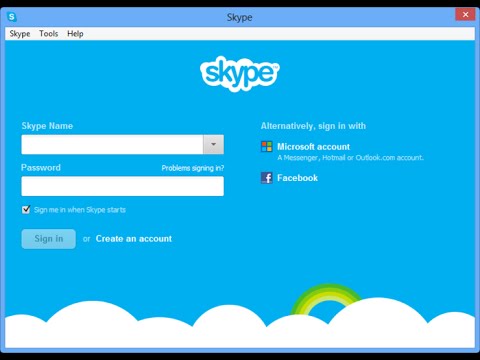The image depicts a Skype login interface with a predominantly blue background. At the bottom of the screen, there are stylized white clouds, whimsically edged, with a small rainbow consisting of yellow and green arcs stretching over part of them. In the upper left corner, the iconic Skype logo, a white "S" within a blue diamond shape, is prominently placed. At the top center, "Skype" is written in black, balanced by a red box with a white "X" on the top right corner.

Right below the banner segment, a white navigation strip is visible, starting from the left with the text "Skype Tools and Help." The central portion of the screen features "Skype" in blue text superimposed on a white cloud graphic. Below this, labeled fields for "Skype name" and "Password" are displayed, both within white data entry boxes. To the right of the password field, there's a prompt reading "Problem signing in?" followed by a checkbox labeled "Sign me in when Skype starts," which is ticked with a black checkmark.

Further down, options for "Sign in" or "Create account" are listed. Additional login alternatives are offered beneath, instructing users they can "Alternatively sign in with Microsoft account, Messenger, Hotmail or Outlook.com account, or Facebook." The color palette of the interface includes various shades of blue, white, red, black, gray, green, and yellow, contributing to the overall visually engaging design.